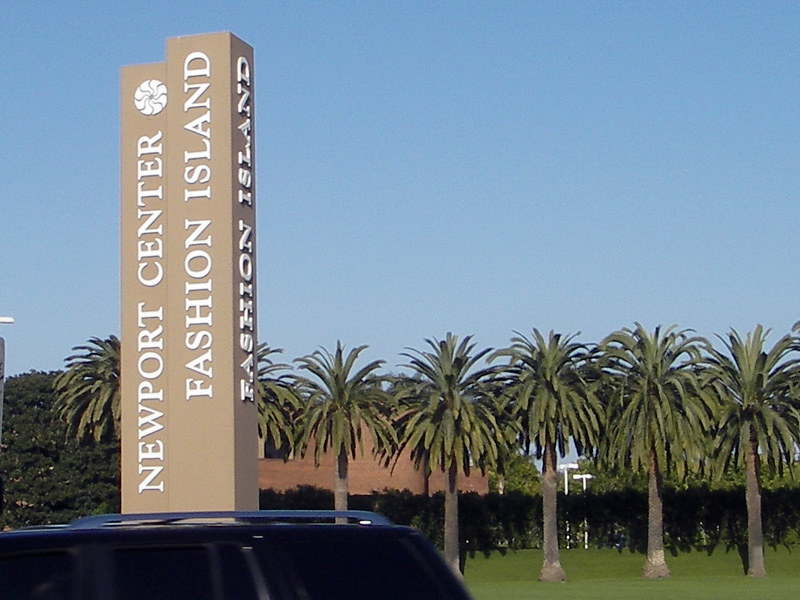The image portrays a clear, bright blue sky, without a single cloud, suggesting it was taken on a perfect day. Dominating the background is a precise line of at least five tall, identical palm trees, equally spaced. They stand on a well-maintained expanse of vibrant green grass. There are additional palm trees at the edges, indicating a probable total of seven. Located behind the trees, a red brick building is visible, along with two white, cross-like objects. The bottom of the photo captures the top portion of a dark-colored SUV with dark windows and a silver luggage rack. To the left of the image, two towering tan-colored signs are prominently visible with white text reading "Newport Center, Fashion Island." The same text appears on the side of the sign that faces the opposite direction. The scene is further softened by more trees and shrubbery in the backdrop, framing the setting in a picturesque outdoor environment.